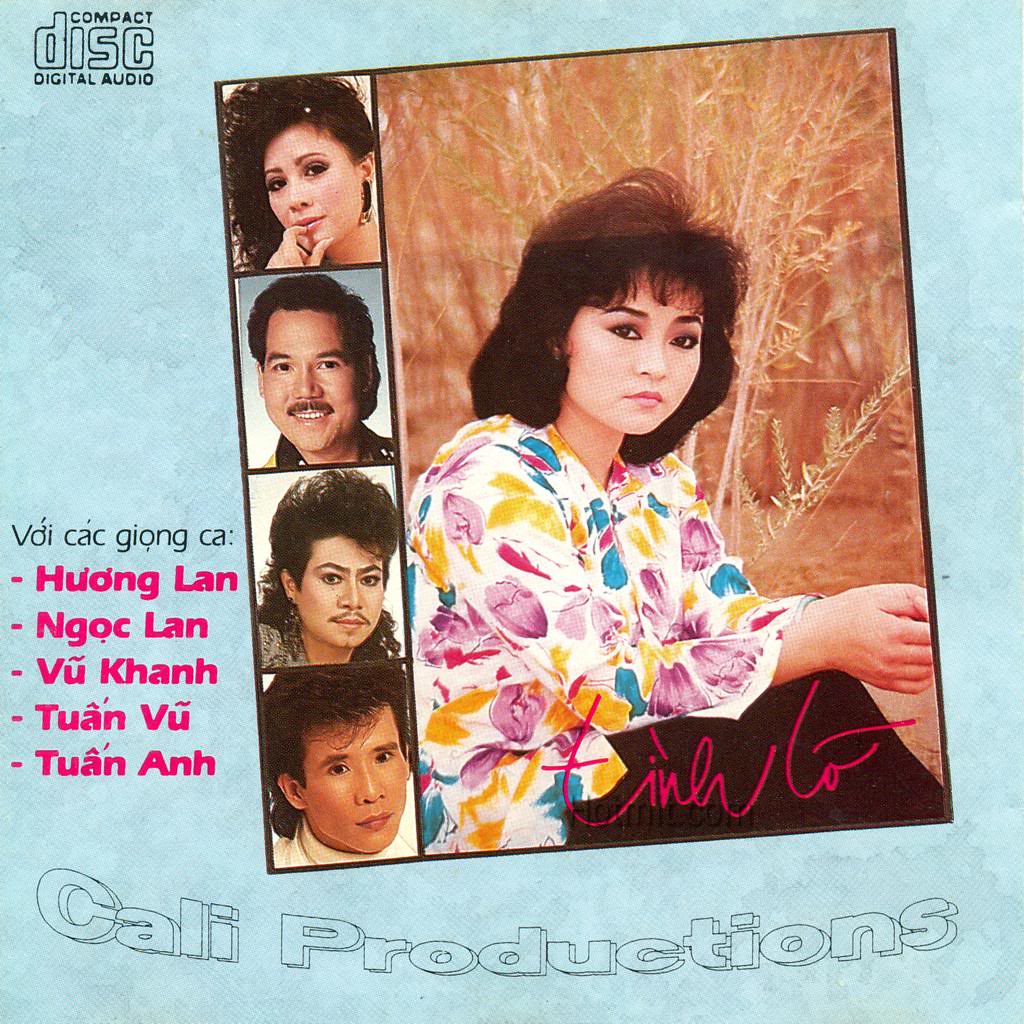The image depicts a music CD cover with a light blue background. In the top left corner, it features the text "Compact Disc Digital Audio." Dominating the center of the cover is a prominent image of an Asian female artist wearing a floral shirt and black pants. To the left of her image, there are five rows of text in a different language, written in pink. Centrally aligned alongside her image, there are smaller square pictures in a vertical arrangement of various Asian artists. The cover also showcases a palette of colors including light blue, black, purple, pink, white, yellow, and teal. At the bottom of the image, the text "Kali Productions" is displayed, providing a finishing touch to the detailed and vibrant album cover.